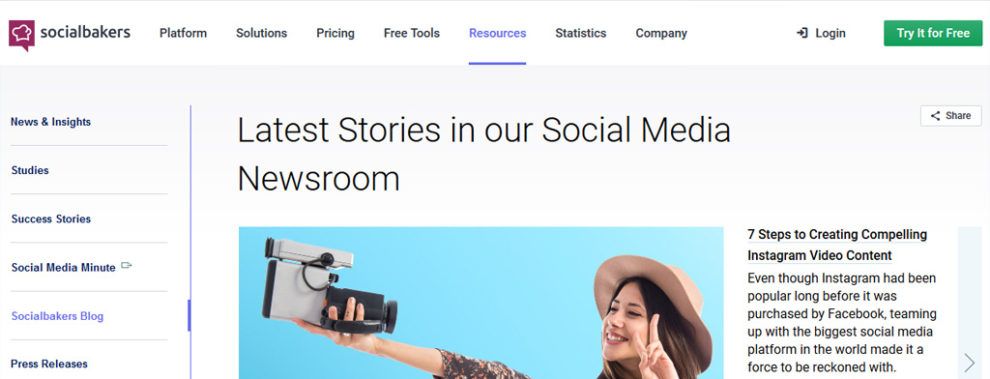Here's a cleaned-up and detailed caption for the image described:

"The image showcases a screenshot from the Social Bakers website. The navigation bar at the top includes tabs labeled 'Platform,' 'Solutions,' 'Pricing,' 'Free Tools,' 'Resources,' 'Statistics,' 'Company,' 'Login,' and a prominent green banner reading 'Try it for Free.' The 'Resources' tab is highlighted in blue, indicating it is the active selection. 

On the left-hand side of the page, there is a vertical menu with options such as 'News and Insights,' 'Studies,' 'Success Stories,' 'Social Media Minute,' 'Social Bakers Blog,' and 'Press Releases.' The 'Social Bakers Blog' tab is currently selected.

In the main content area, the headline reads 'Latest Stories in Our Social Media Newsroom.' Below the headline is an image of a Caucasian woman holding a video recorder extended in her right hand, capturing a selfie video. She flashes a peace sign with her left hand. Adjacent to this image, text reads: 'Seven Steps to Creating Compelling Instagram Video Content.'"